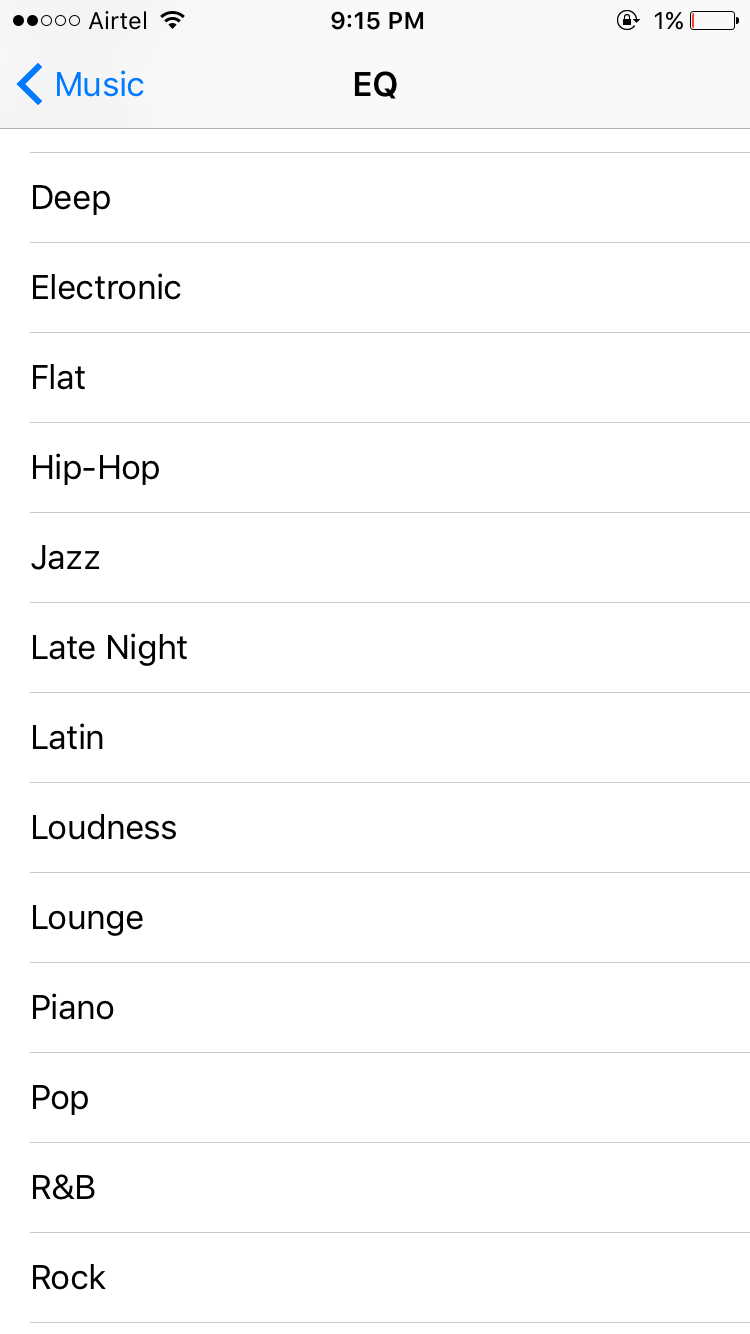A detailed caption for the screenshot of the mobile application:

"The image is a screenshot taken from a mobile device displaying an application interface. At the top of the screen, the device status indicators are shown. The mobile network signal, provided by the carrier 'Airtel,' is indicated by two circles. The Wi-Fi signal is full, indicating a strong connection. The current time displayed is 9:15 p.m. Next to the time, a lock icon is visible, suggesting the device is locked. The battery life is critically low at 1%, highlighted by a red, nearly exhausted battery icon. 

On the left side of the screen, a navigation arrow in blue font points to the left, adjacent to the word 'Music.' At the top of the app interface, the label 'EQ' is displayed, indicating the Equalizer settings. Various equalizer presets are listed below, including 'Deep,' 'Electronic,' 'Flat,' 'Hip-Hop,' 'Jazz,' 'Late-Night,' 'Latin,' 'Loudness,' 'Lounge,' 'Piano,' 'Pop,' 'R&B,' and 'Rock.' The application interface features a clean design with a white background and black font for the text, making the options easy to read."